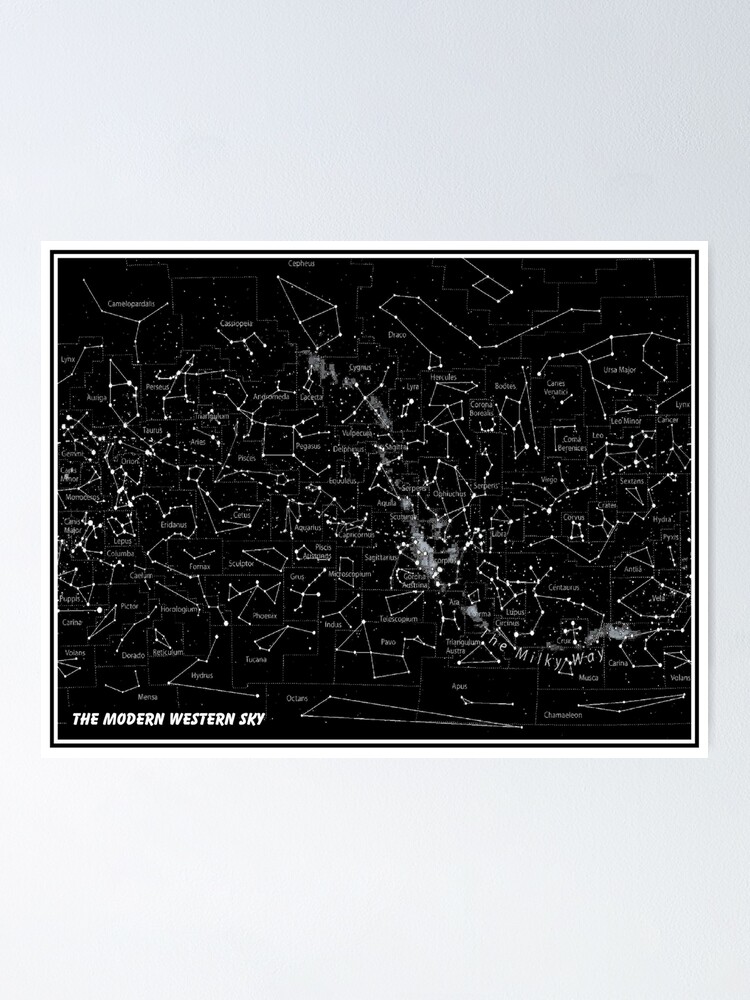The image features a square, vertically aligned, framed picture set against a light gray wall, which fades to a paler gray at the bottom. The frame consists of a white outer edge, a black inner border, and another white line, creating a sleek, modern presentation. The central artwork is predominantly black, speckled with numerous tiny white dots representing stars. Among these, various star constellations are depicted with lines connecting the stars, forming geometric shapes and symbols. Prominently labeled in the lower left-hand corner in white capital letters on a black background is “The Modern Western Sky.” Within the map, the Milky Way is clearly indicated, and you can also find recognizable constellations like Orion's Belt, Sagittarius, Leo, Hydra, and the Big Dipper, although the smaller text detailing each constellation is difficult to read.